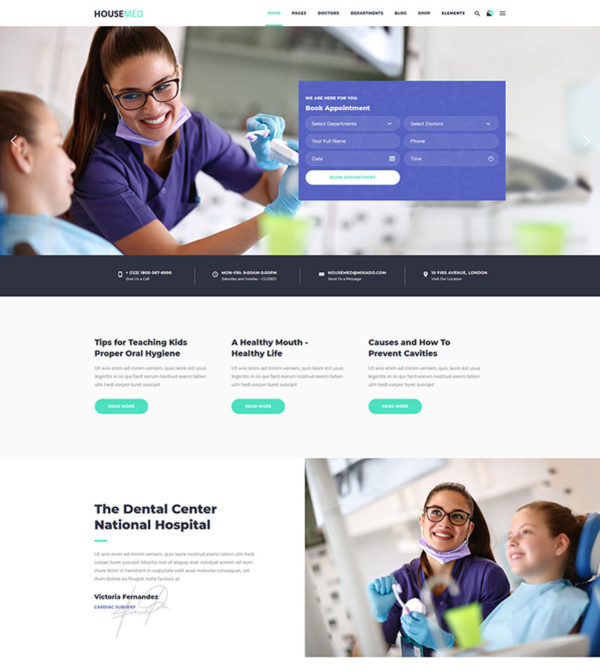Top image: A woman dressed in a purple outfit, likely a dentist or dental hygienist, is smiling warmly. She wears a mask pulled down beneath her chin and has glasses on. Her dark hair is tied back in a ponytail. She directs her attention to a patient on her left, whose partially visible face is accompanied by a blue garment, typical of a dental setting. Above this scene, the words "House" (in black) and "Med" (in light blue) appear. A purple box with the text "Book Appointment" and clickable arrows for date and time selection is also displayed. Below this, in black text, it reads "Dental Center National Hospital."

Bottom image: The same dental professional is now looking upward, as if focused on a screen in front of her. She wears blue plastic gloves and holds a toothbrush or dental cleaning tool in her hand. To her side, a younger girl patient wears a blue protective apron, standard for dental procedures. A green cup is placed on the patient's right side.